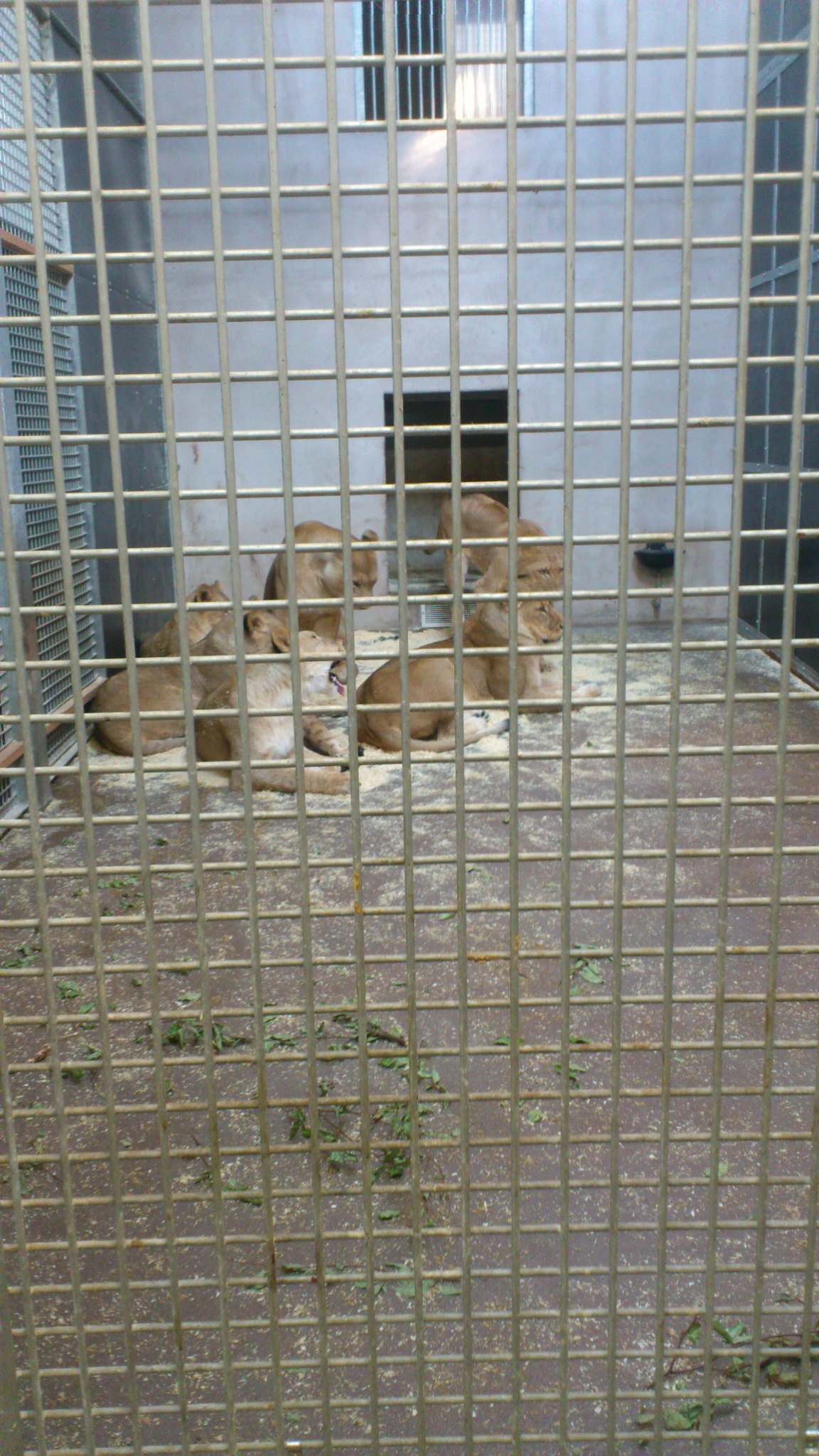In this photograph, we observe a group of five young lionesses huddled together, all lying down and appearing relaxed. They gaze intently towards the right side of the image. They are enclosed within a tall, reinforced steel cage, designed to ensure safety both for the humans outside and the lions inside. The cage's structure features repeating metal bars that prevent any interaction that could cause harm.

The ground inside the cage is a mix of light tan stone and soil scattered with small patches of green vegetation. Surrounding them is a tall, white building with metal guard bars over its windows, likely functioning as an additional measure to protect the lions. This building has a square doorway through which one of the lionesses appears to be re-entering, suggesting that the enclosure consists of multiple connected areas. The background displays a large, gray wall, adding to the enclosed feel of the space. Despite the confines, the lions seem at ease, physically close and comfortably resting on the sandy terrain.